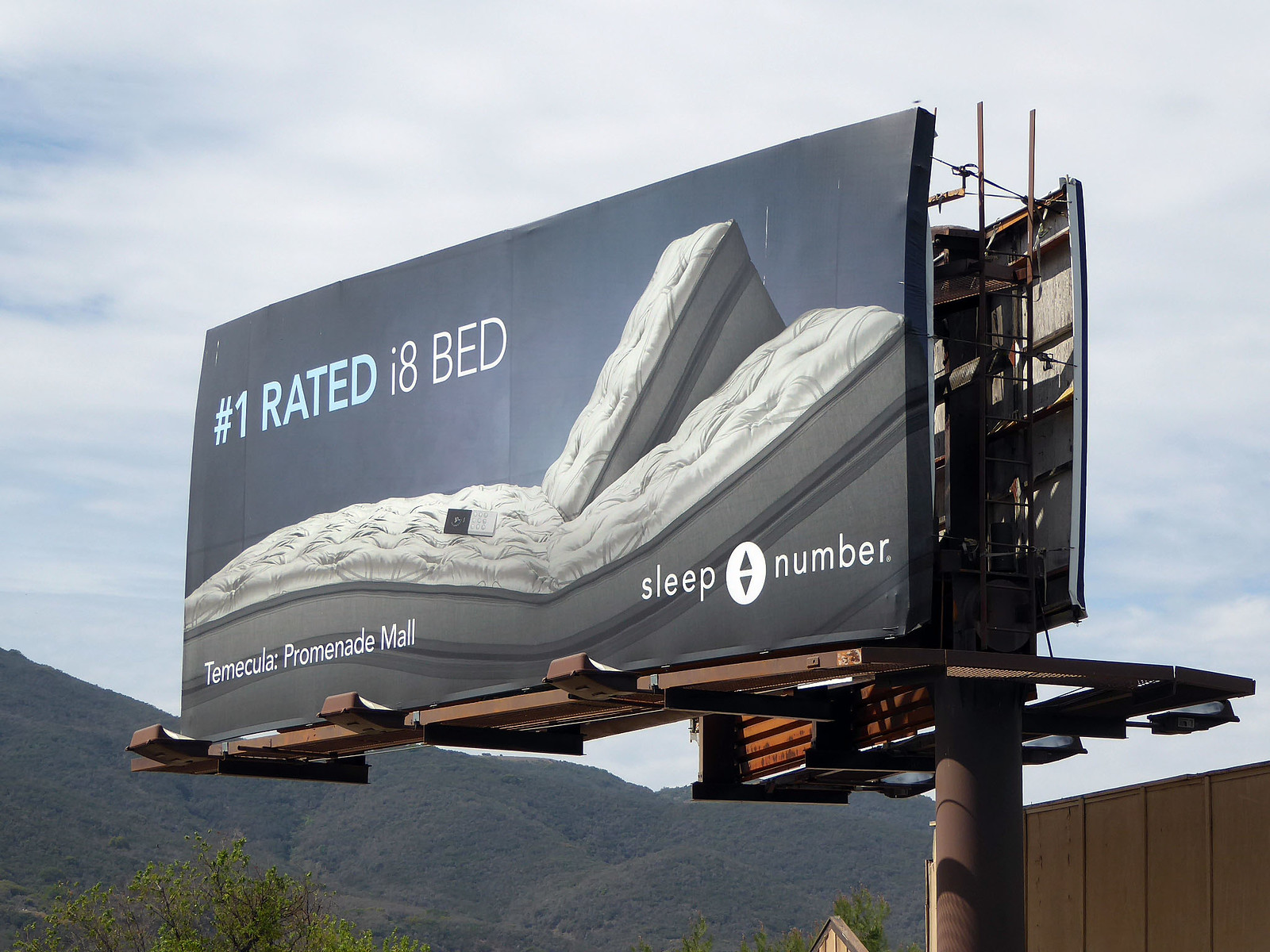This outdoor photograph features a prominently placed billboard set against a backdrop of partially blurred gray and brown mountain ranges, which decrease in height from left to right. The blue sky above is dotted with wispy clouds, hinting at a pleasant day. A tall brown wooden fence occupies the bottom right corner, contrasting with the landscape. In the middle of the image, mounted on a substantial rust-colored cylindrical metal post, the billboard is angled diagonally with its right side closer to the viewer.

Two billboards are visible on the sign structure: the main billboard, displayed clearly, and another partially obscured one on the right. The main billboard advertises a high-rated mattress with a split design, allowing each side to be individually adjusted, as indicated by the graphic depiction of the mattress's back part lifted up. The text on the billboard reads: "Number One Rated I-8 Bed," followed by "Temecula Promenade Mall." In the lower right corner, the term "Sleep Number" is displayed alongside up and down arrow graphics, symbolizing adjustable settings. The mountains, trees, and billboards combine to suggest a rural setting for this advertisement.